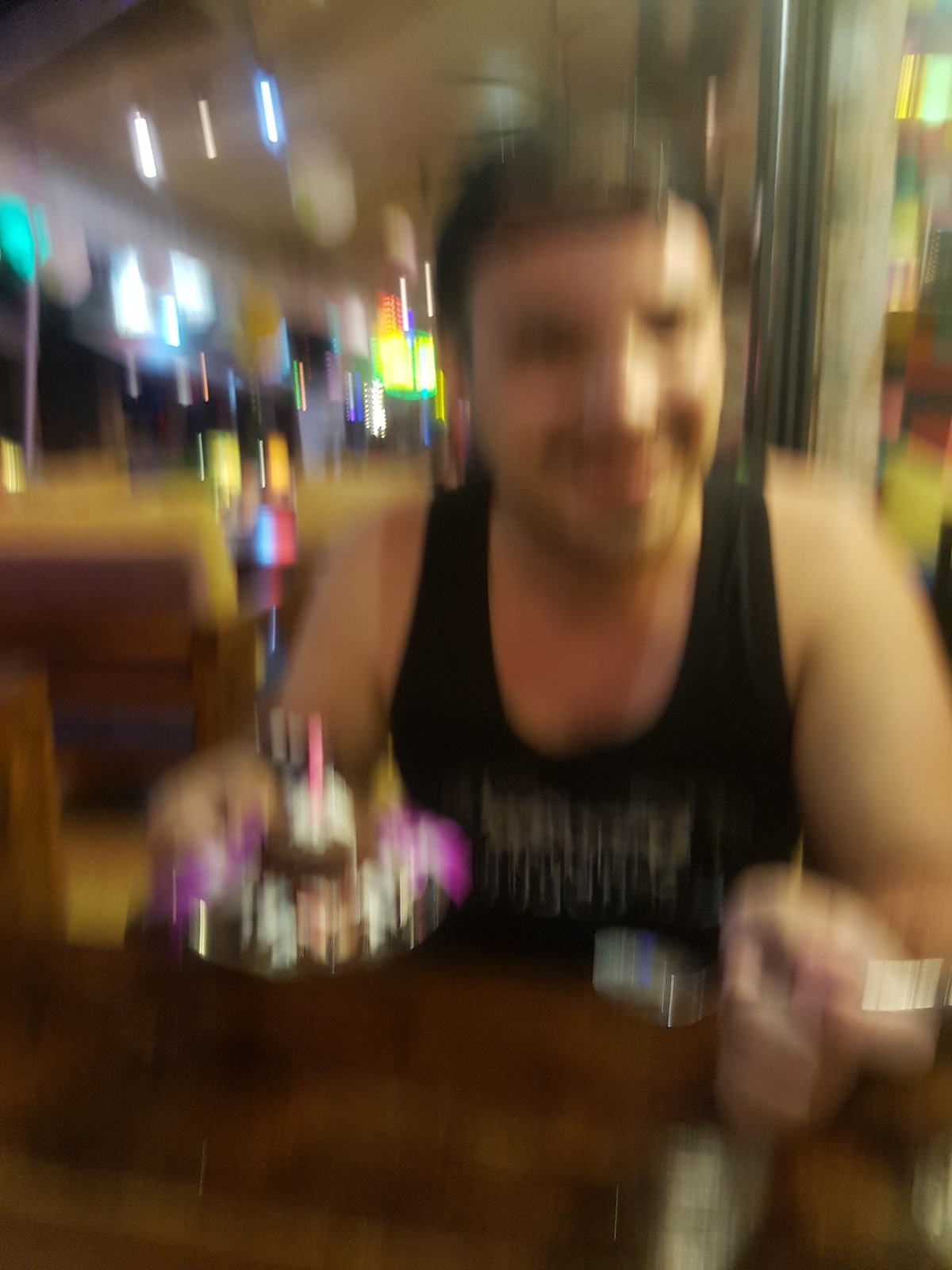The extremely blurry photograph depicts a light-skinned male, possibly in his 20s or 30s, with light brown hair, a mustache, and a beard, sitting in a booth at a bar or an eating establishment that features colorful neon lights in the background. He is smiling and wearing a black tank top with some sort of white or yellow writing on it. In his left hand, he holds a utensil—likely a fork or spoon—while his right hand cradles a vibrant, colorful dessert that includes shades of purple, pink, white, and red, which might be a celebratory dish such as a birthday cake or ice cream. The man is seated at a narrow brown table, possibly next to a window, giving the impression of a long but narrow space. The overall scene suggests a joyful moment of celebration, despite the blurriness of the image.